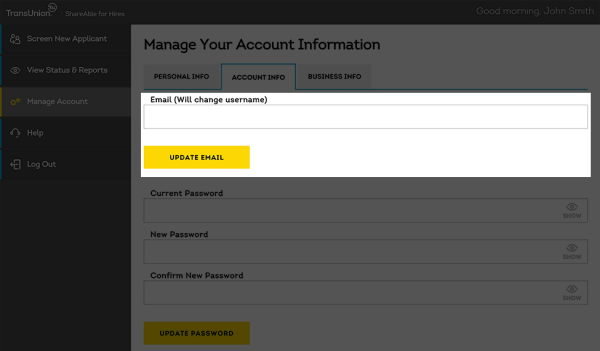A detailed caption of the image:

The screenshot captures a user interface that appears to be from a web application, viewed on either a laptop or a tablet. The top section features a black banner extending across the entire width of the screen. Despite its faded nature, the banner contains several white text elements: "trains a union," "screen new applicant," "view status and reports," and "manager counts," with the last element highlighted in gray. Additionally, there are options for "help" and "log out" on the right side of the banner. In the top right-hand corner, it faintly displays the greeting "Good morning, John Smith."

Beneath the banner, the main background is white but also somewhat faded. The phrase "manage account information" is prominently displayed in black font. Below this phrase are three tabbed sections: "personal info," "account info," and "business info." The "account info" tab stands out with a blue outline indicating it is the active tab.

Central to the interface is a distinctly visible white box containing fields for updating account details. The label "email" is shown in black font with a note in parentheses stating "(will change username)" followed by a thin input box for the email address. At the bottom right of this section, a yellow rectangular button with black text reads "update email."

Subsequently, there are three input fields for password management: "current password," "new password," and "confirm new password," each labeled in bold black letters. At the bottom of this section, a yellow rectangular button, similar to the email update button, reads "update password."